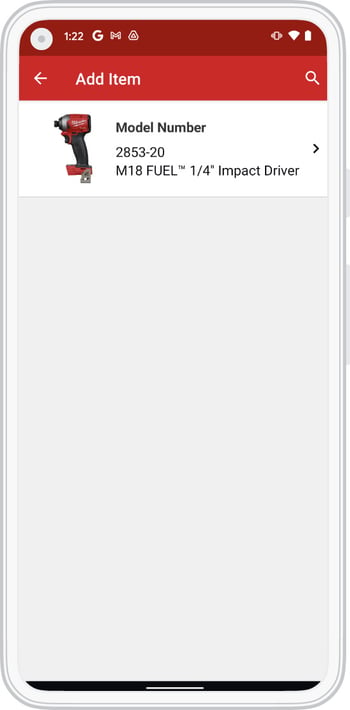A digital rendering of a white cell phone is displayed on the screen, with intricate details resembling a computer-generated image. The phone is adorned with a red strip at the top, transitioning from a darker shade on the left to a lighter shade on the right. In the darker red section, it displays various status indicators: "122" followed by letters "G" and "M," and a triangle icon. The right side of the red strip shows a vibrate icon, a Wi-Fi icon, and a full battery icon. 

Below the red strip, in a lighter red area, there are actionable icons: a red arrow pointing left with the label "add item" on the left side, and a search icon on the right. Both labels and icons are in white font.

Taking up approximately a fourth of the screen below the red strip is an image of what appears to be a drill. This image is accompanied by text in white font stating "model number 2853-20" and "M18 FUEL™ 1/4 inches impact driver," followed by a right-facing arrow.

The remaining three-fourths of the screen features a plain white background, with a thin black strip positioned at the bottom. The overall composition presents a clean and structured layout, with a distinct dichotomy between the red, white, and black elements.